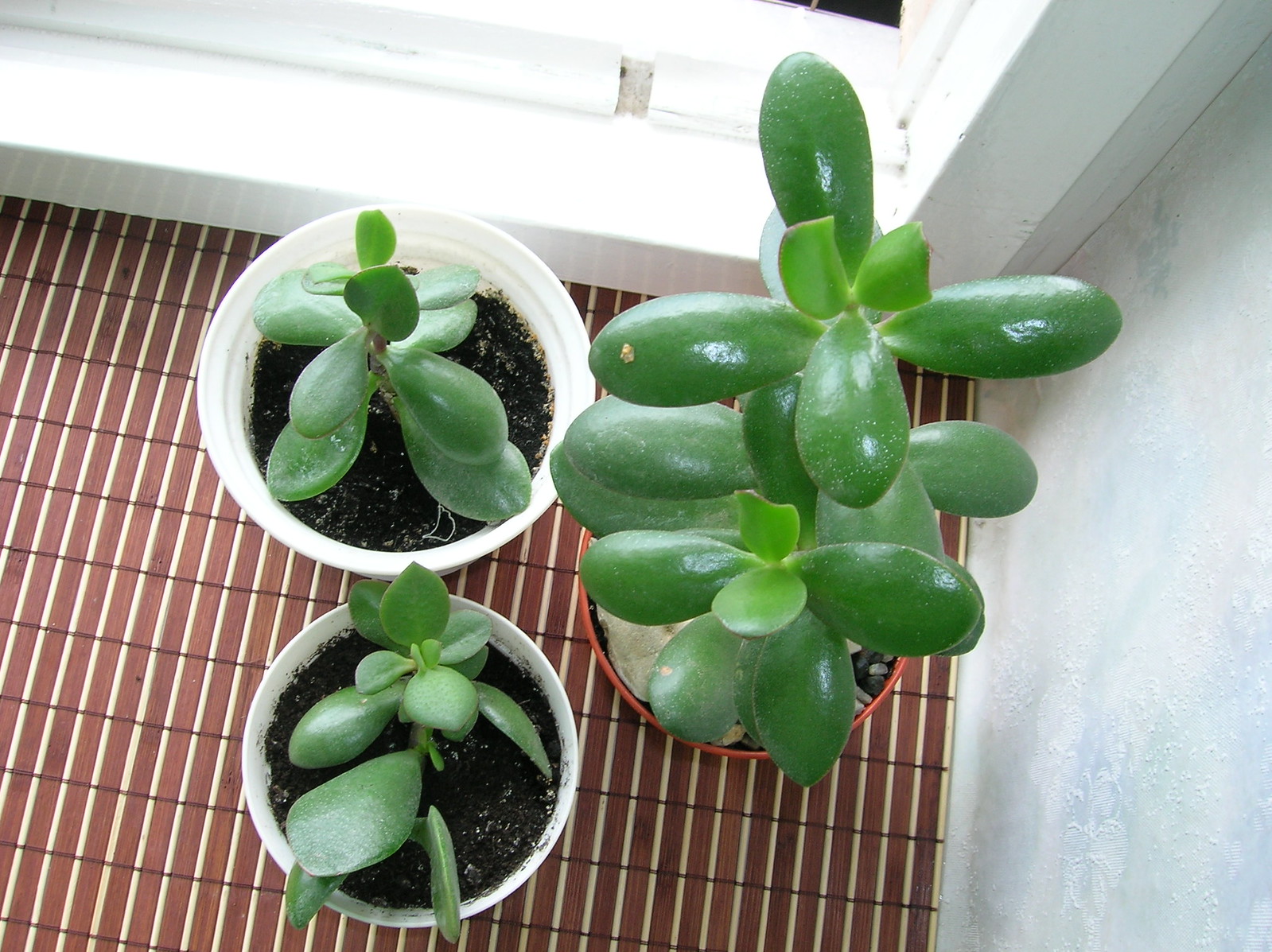The photo captures a top-down view of three jade plants, or succulents with fleshy leaves, arranged on a stone-like surface near a bright white-framed window. The surface features a stone texture with horizontal grooves and vertical white stripes, contributing to a neat appearance. To the right, there's a white textured wall. The scene is brightly illuminated by natural sunlight streaming through the window, suggesting the plants are intentionally placed to benefit from the light. 

To the right, a larger, more mature jade plant sits in a brick-colored (or orange) pot with black soil interspersed with white specks, possibly decorative rocks. This plant exhibits multiple layers of leaves forming cross shapes, with newer, smaller light green leaves at the top. To the left, two smaller jade plants grow in white pots, their dark, slightly moist soil sprinkled with tiny white specks. The leaves of these smaller plants are rounded and plump, indicating they are well-watered and healthy. Overall, the detailed arrangement and bright setting highlight a nurturing environment for these thriving houseplants.